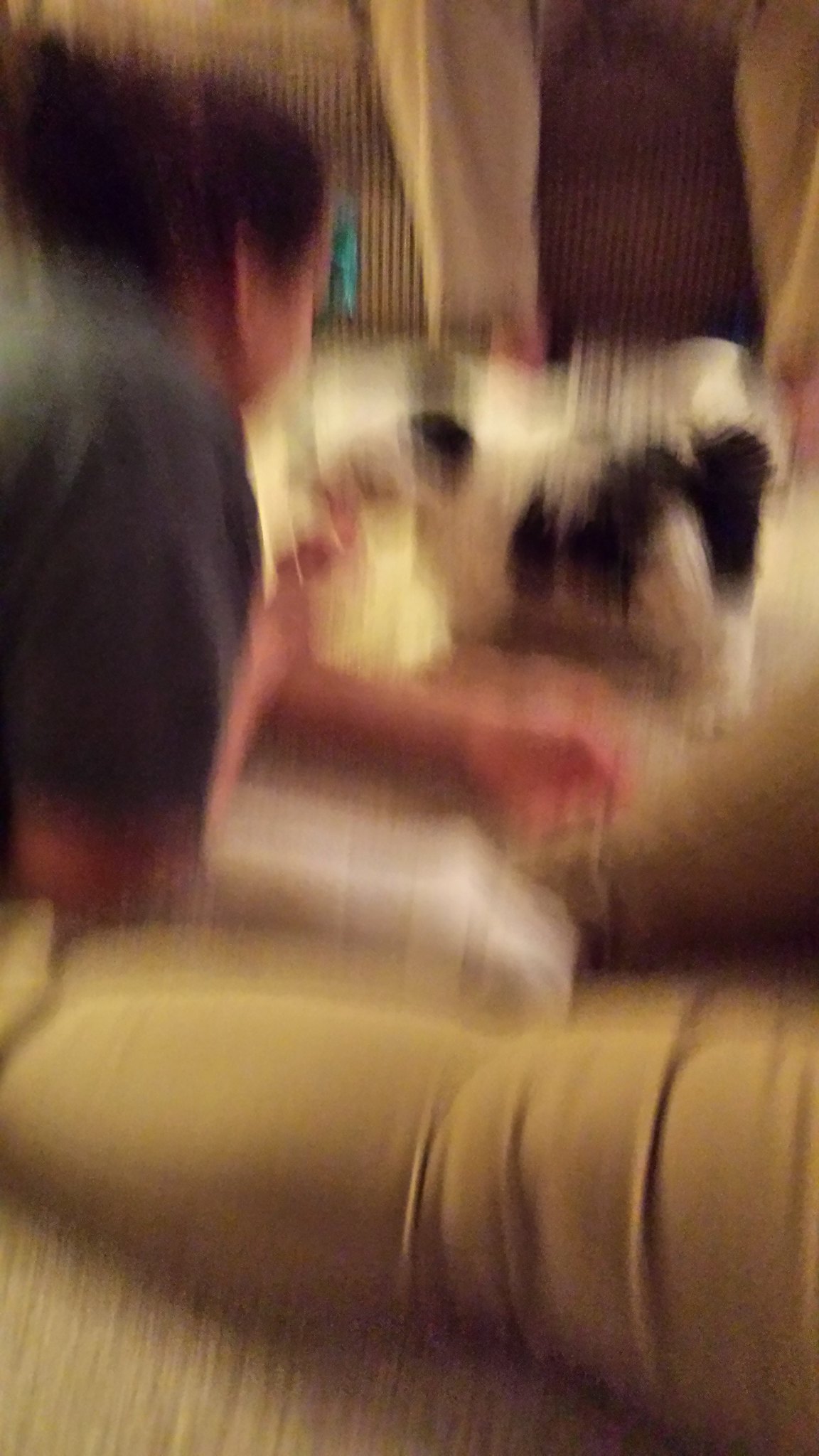The image is a very blurry, vertically-oriented photograph, likely captured while in motion, resulting in its out-of-focus nature. At the bottom of the image, there's a tan cushion, possibly from a couch or chair. Just above it, a person's leg is visible; the leg appears larger and is clad in tight, tan yoga pants, with the calf and thigh extending from left to right across the frame. In the upper left-hand corner, a young Caucasian girl with long brown hair tied back is prominently featured. She is wearing a dark blue-green t-shirt and is engaging with a small, shaggy black and white dog, which has black ears, black spots, and a tail. The dog is very tiny, around 10 pounds. The girl is partially laying down, propped up on her left arm while her right hand reaches out towards the dog, possibly holding a small yellow item. Surrounding the dog, two other people's legs are noticeable—one in brown pants and the other in khaki beige pants. In the background, there are more tan shapes and a somewhat rectangular black shape, though the overall image remains very fuzzy and difficult to parse clearly due to its poor focus.